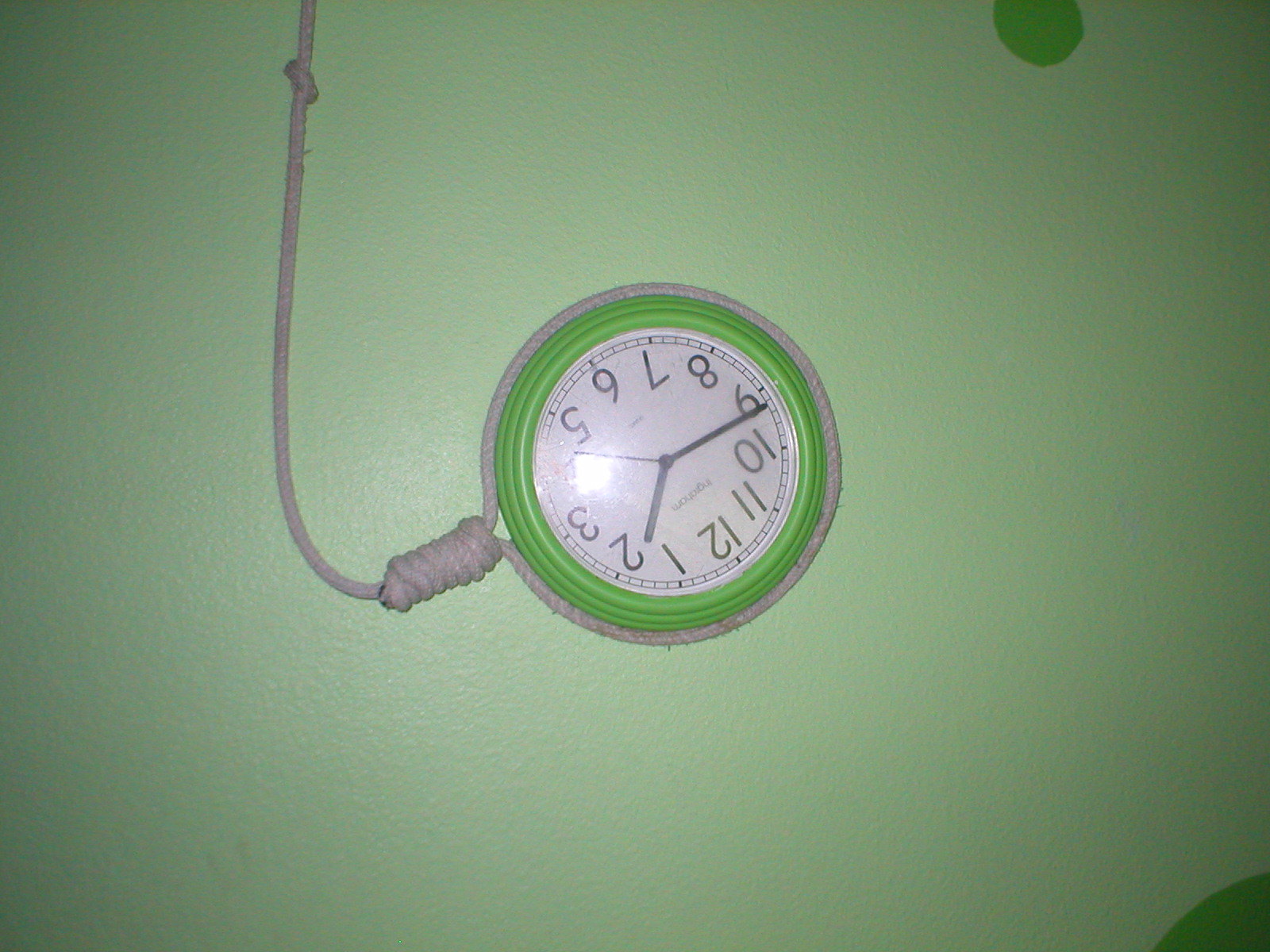The photograph showcases an old-style plastic clock prominently centered on a spring green wall adorned with a few darker green polka dots. The clock, a darker shade of green reminiscent of summer grass, is intriguingly tilted so that the numeral "1" occupies the position typically held by the numeral "6." This unconventional placement hints at an artistic or symbolic intent. The clock, displaying the time as approximately 1:45, features a clear face framed by a white rope fashioned into a noose that ascends along one side, adding a provocative and possibly symbolic touch to the composition. The striking green of the wall contrasts vividly with the clock, enhancing its visual impact and suggesting a deliberate, thought-provoking design.